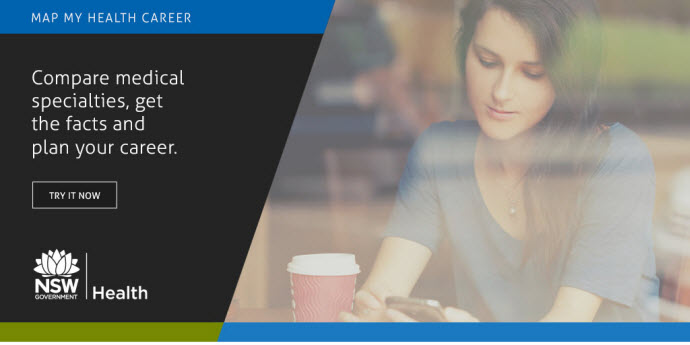The image is an advertisement, possibly part of a website, showcasing a young woman engrossed in her smartphone, with her head tilted down as she scrolls. To her right is a disposable coffee cup, suggesting a casual, everyday setting. The scene appears to be viewed through a window, indicated by a blurry reflection that includes a possible street or car, adding depth and context to the background.

On the left side of the image is the promotional content. At the top, there's a horizontal blue line with the text "Map My Health Career" in white font. Below this, a black, unusually-shaped upside-down trapezoid features the message: "Compare medical specialties, get the facts, and plan your career." Enclosed within the trapezoid is a call-to-action button labeled "Try it now."

At the bottom of the promotional section, an icon of a lotus flower is displayed, followed by the words "NSW Government." A horizontal line separates this text from the word "Health." Completing the design, an olive green bar transitions into the same dark blue color seen at the top, extending beneath the image of the woman.

The overall composition creates a compelling and informative advertisement aimed at guiding users towards planning their careers in the medical field.